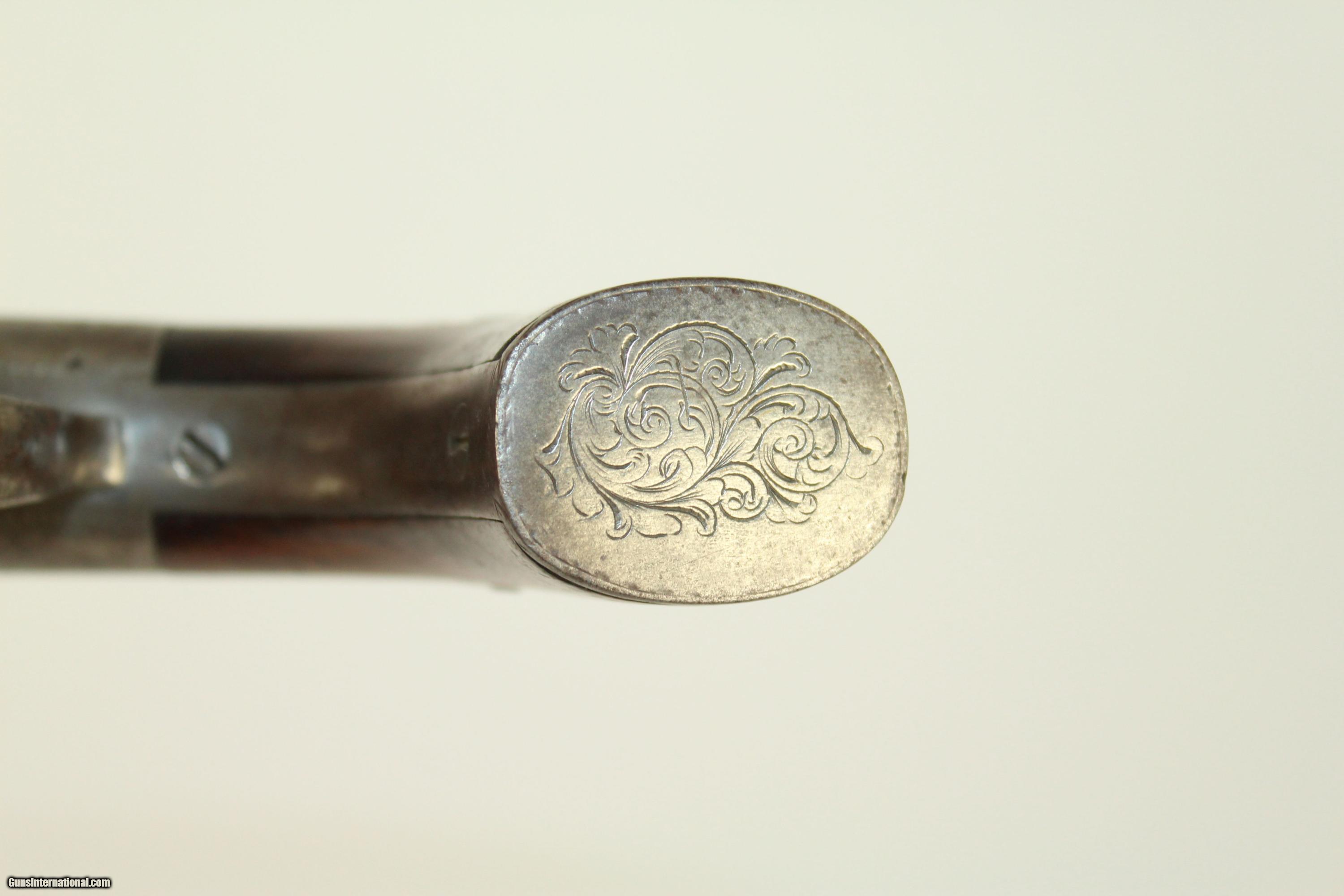The image depicts the intricately detailed butt of a revolver, set against an off-white, slightly beige-grey background with a black shadow overlaid on the bottom left corner, where the text "gunsinternational.com" is visible. The visible part of the gun is predominantly composed of tarnished silver and wood. The silver section features an ornate, swirly design with ridges and intricate patterns resembling clouds or water waves swirling towards the center. The wooden part of the gun extends downward, showing a varnished silvery-brown hue that might appear darker due to shadowing. Additionally, a screw is visible, suggesting a point for maintenance or assembly. The overall craftsmanship of the revolver's butt is highly detailed and ornate, reflecting a blend of both functional and decorative elements.